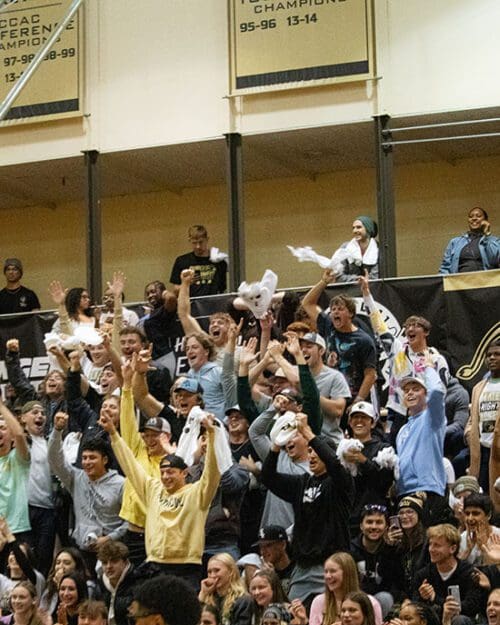The image depicts an energetic crowd of predominantly young fans, likely high school or college-aged, gathered at an indoor sporting event. The scene captures a moment of celebration; many fans are standing with their hands raised, visibly cheering for a favorable outcome. In the background, there are banners displaying years such as "97," "98," "99," "95," "96," and "13-14," potentially indicating past championships. The crowd is a colorful mix, with attendees wearing clothing in various hues including yellow, green, black, and white. Some fans don baseball caps, and a few are holding items over their heads, possibly t-shirts, towels, or stuffed animals resembling mascots. A notable figure in the front has both hands raised high, amplifying the joyous atmosphere. The setting appears to be an arena with multi-level seating, and white objects are being thrown into the crowd, adding to the celebratory chaos. The image, taller than it is wide, effectively captures the vibrant, triumphant spirit of the fans at this unidentified sporting event.